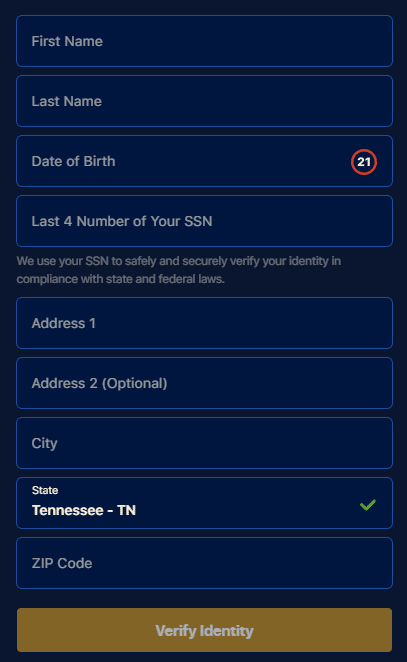This image is a smartphone screenshot featuring a webpage section designed for identity verification. The section initially contains fields for the user to input their first name, last name, date of birth, and the last four digits of their Social Security Number (SSN). Beneath these input boxes, there is a disclaimer stating, "We use your SSN to safely and securely verify your identity and ensure compliance with state and federal laws."

Following this, the form continues with additional input fields for address details, including:

1. **Address Line 1**
2. **Address Line 2** (optional)
3. **City**
4. **State** (indicated as Tennessee-TN with a green checkmark)
5. **ZIP Code**

At the bottom of the form, there is a prominent brown button labeled "Verify Your Identity," which users can press to submit their information for verification. The webpage aims to collect necessary personal details to confirm the user's identity in accordance with legal requirements.